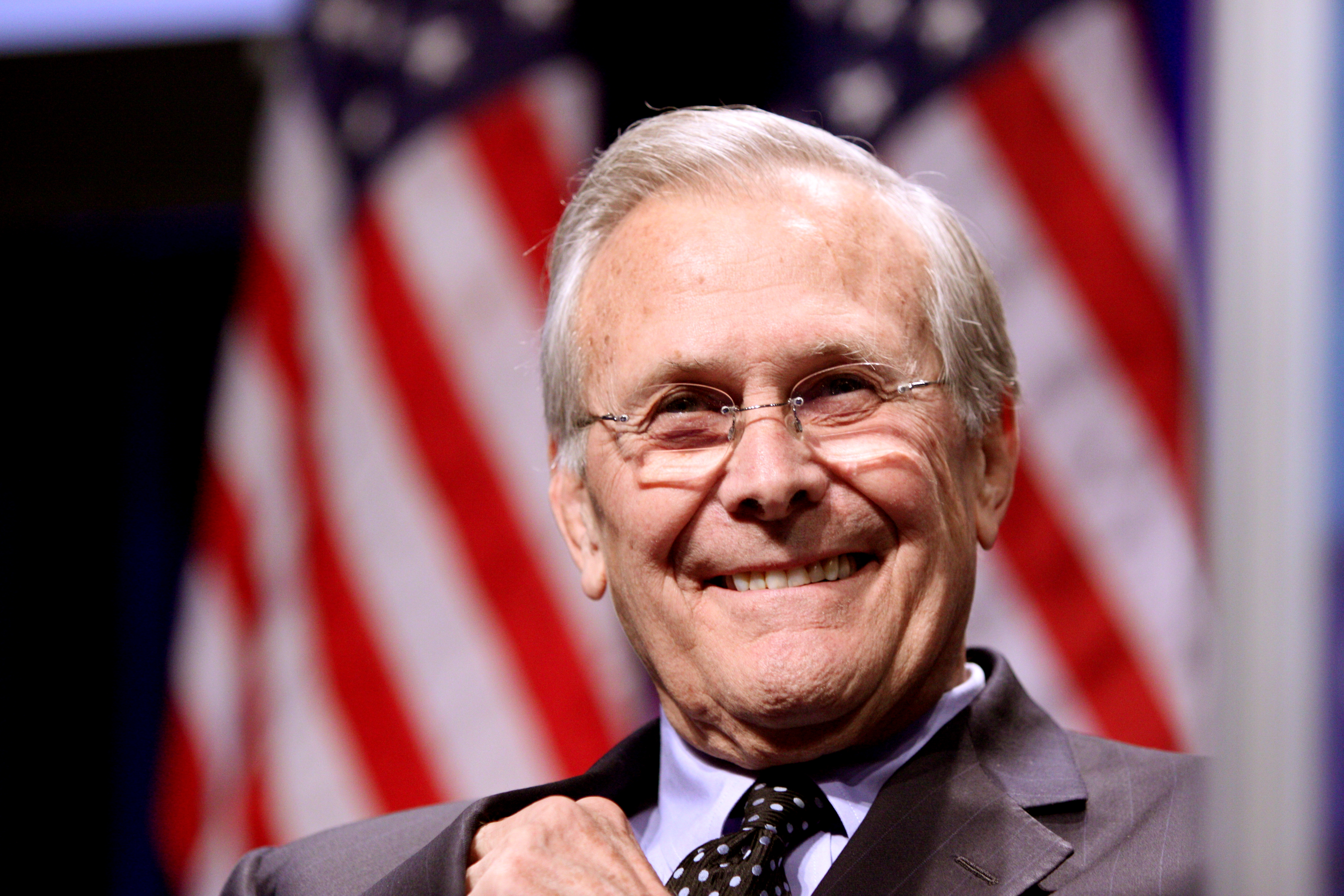This image captures an elderly politician, likely Donald Rumsfeld, posing from the shoulders up amid a formal or public event. His white, slightly patchy hair is neatly groomed, and he dons a pair of frameless, short-lensed glasses. He is smiling warmly, revealing his top teeth. He is dressed in a dark gray suit jacket with fine white lines or checkers, a white collared dress shirt, and a black tie adorned with white polka dots. His left hand is clenched in a fist and held near his chest. In the blurred background, two American flags hang vertically from flagpoles, displaying their red, white, and blue colors. Behind him, there is a dark backdrop, indicative of an indoor setting, possibly a convention or speaking event, as suggested by overhead lighting casting a soft glow on his head.